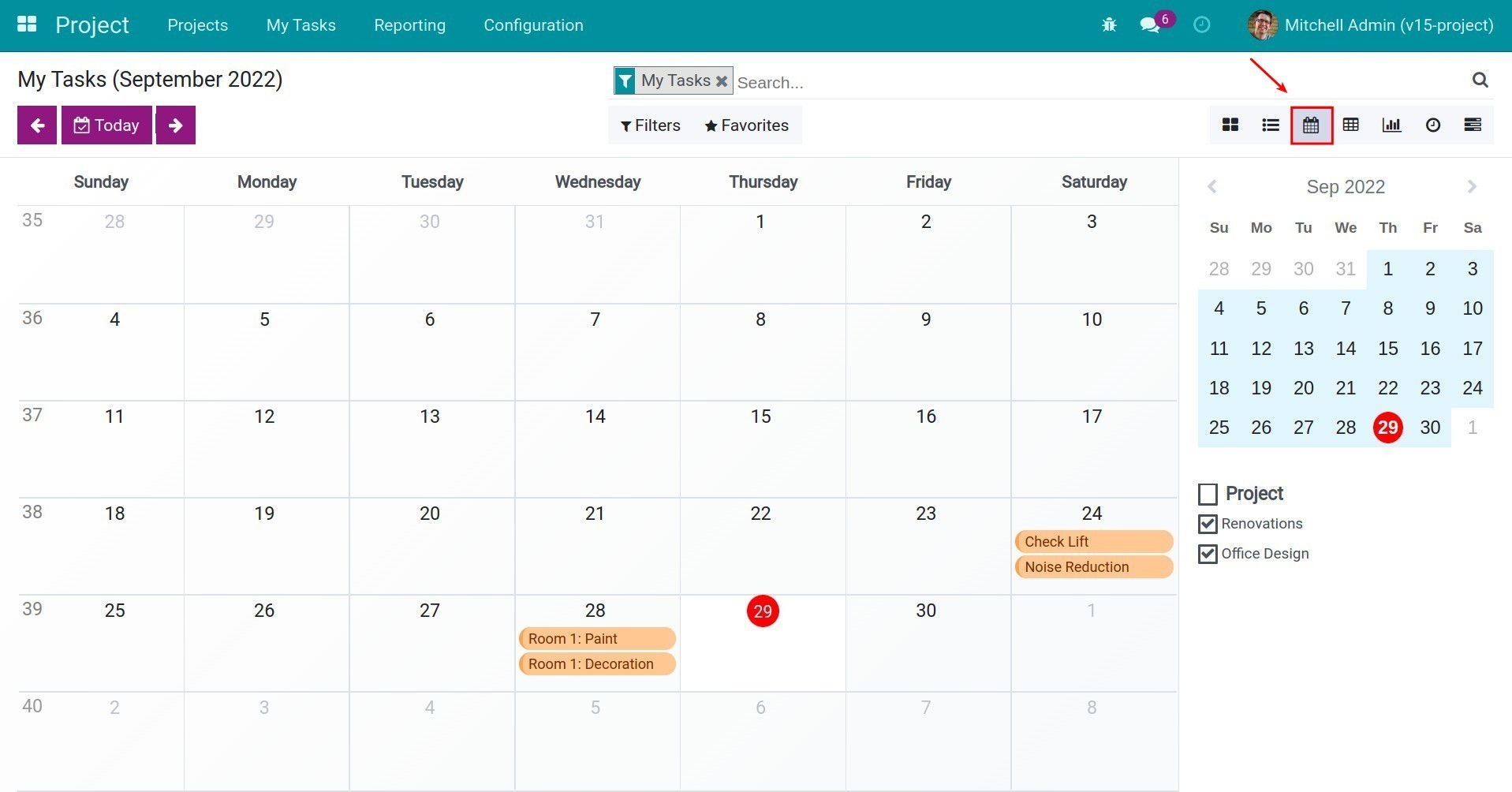The image showcases a detailed project calendar interface. At the top of the interface, there is a green-blue banner featuring the Microsoft logo followed by menu options: "Project," "Projects," "My Tasks," "Reporting," and "Configuration." Adjacent to these, there are three icons and a small photo of a man named Mitchell Edmund, marked under "V15-Project."

Below the banner, the section reads "My Tasks," dated September 2022, with a search bar nearby. The next line features a purple background labeled "Today" in white letters, alongside options for "Filters" and "Favorites."

The main calendar spans from Thursday, the 1st, to Friday, the 30th. A notable red highlight appears on Thursday, the 29th. Additionally, specific tasks are noted on the calendar. For instance, on Wednesday, the 28th, tasks include "Room 1 - Paint" and "Room 1 - Decoration." On Saturday, the 24th, tasks listed are "Check Lift" and "Noise Reduction."

On the right side of the interface, a smaller calendar is displayed, over which seven icons are positioned at the top. Towards the bottom of this smaller calendar, there are two marked project boxes: "Renovations" and "Office Design," both with checkmarks indicating their status.